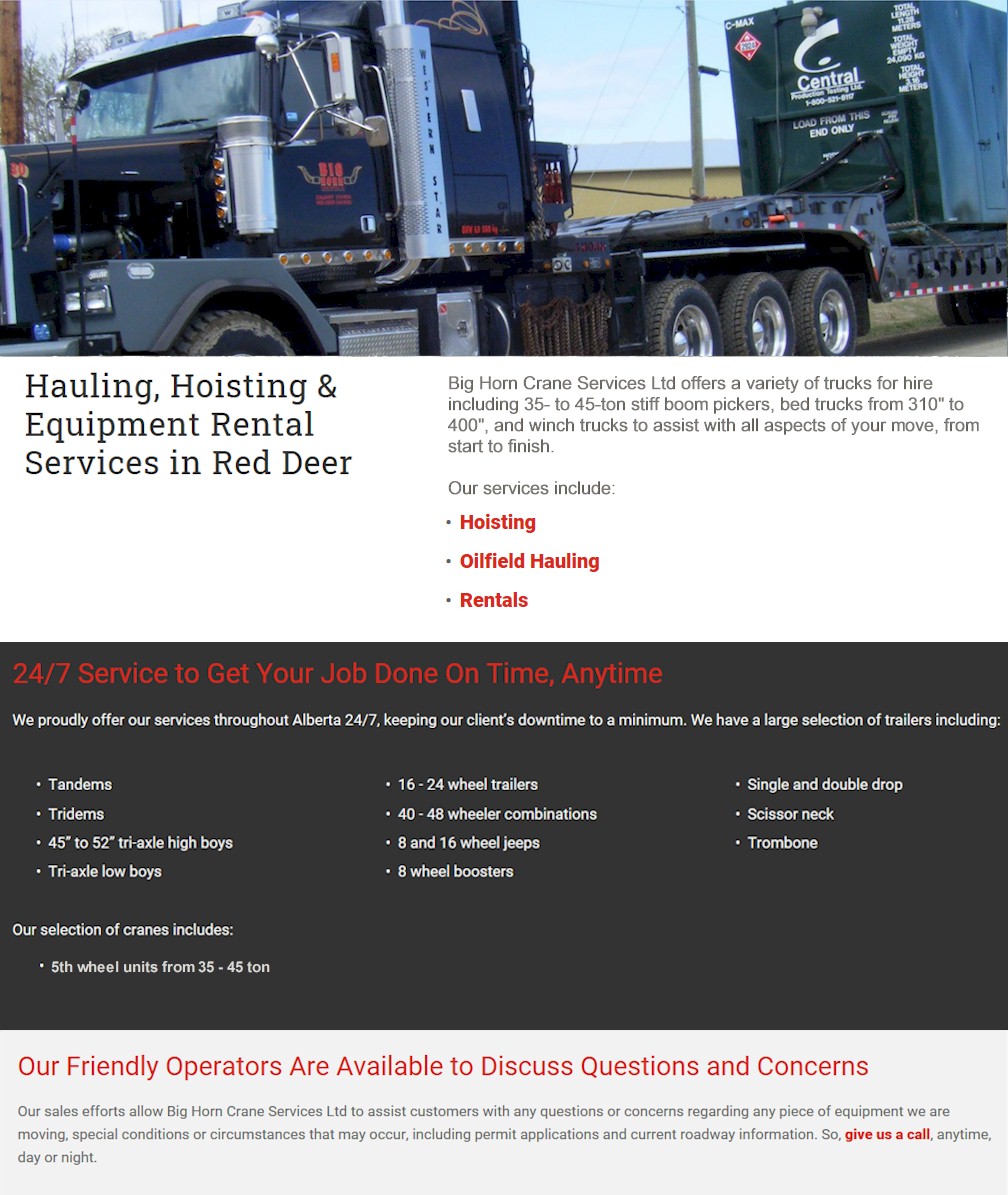The image depicts a white page with marketing content for Big Horn Crane Service LTD. Central to the image is a photograph of a blue truck hauling a large trailer with green sides. The trailer prominently displays the text "Central Product Testing LTD" in white font, alongside a phone number.

Below the photograph, the text reads: "Hauling, hoisting, and equipment rental services in Red Deer. Big Horn Crane Service LTD offers a variety of trucks for hire including 35 to 45-ton stiff boom pickers, bed trucks ranging from 310 to 400 tons, and winch trucks to assist with all aspects of your move from start to finish. Our services include hoisting, oil field hauling, and rentals. We offer 24-7 service to ensure your job is completed on time, anytime. We proudly offer our services throughout Alberta 24-7, minimizing our clients' downtime."

The section continues with an outline of their extensive selection: "We have a large selection of trailers and cranes, including fifth wheel units from 35 to 45 tons." The page also highlights the availability and friendliness of their operators, noting: "Our friendly operators are available to discuss questions and concerns."

The design of the page features a predominantly white background with black text, complemented by sections of gray background with white and red text for emphasis.